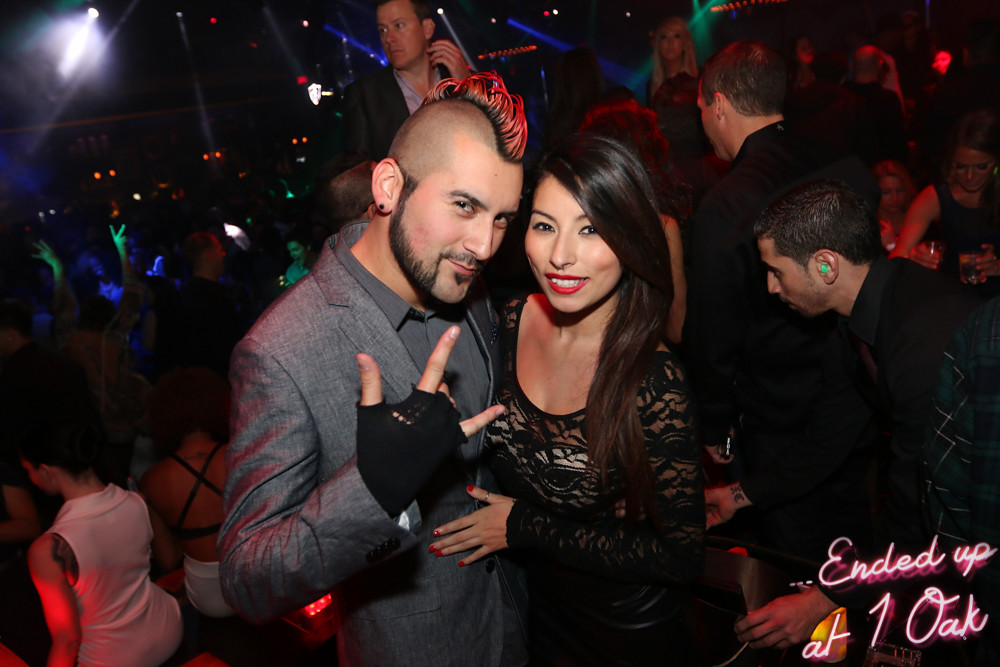In the image of a bustling nightclub interior, the vibrant scene is characterized by swirling blue, green, and red party lights emanating from the upper left and right corners. The crowd appears fairly packed, with young, well-dressed individuals engaging in the nightlife. Dominating the foreground, a striking couple draws attention: the man on the left sports a vivid red mohawk with the rest of his head shaved, a black beard, and mustache. He's dressed in a sleek gray suit coat with a gray shirt beneath and wears a black fingerless glove on his right hand, which he holds to his chest in a classic rock gesture. Beside him, the woman with long black (or possibly brown) hair cascading past her shoulders wears a stylish black lace top, accentuated by her red fingernails and pink lipstick. She smiles warmly at the camera. The ensemble of black, white, blue, green, and pink hues further enhances the lively atmosphere. Scattered details like a man with a green earplug and another individual flashing a peace sign add to the scene’s dynamism. Notably, the phrase "ended up at 1 OAK" glows in neon in the bottom right corner, solidifying the location’s exclusive and trendy vibe.